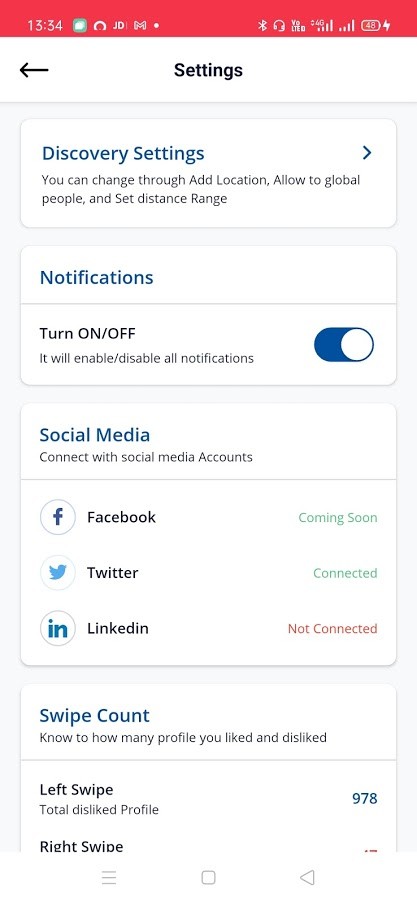The image shows the settings screen of a smartphone, depicted in detail. At the top is a red status bar, which is unusual. The current time is displayed in military format as 13:34. Bluetooth headphones are connected, the phone is charging (indicated by lightning bolts), and there are icons for Wi-Fi and signal strength.

The background is white, with "Settings" written in black at the center and a left arrow icon nearby. Below that, there's a large white box with "Discovery Settings" written in blue, followed by black text explaining you can change ad location, allow visibility globally, and set a distance range. Another white box below has "Notifications" in blue, with a description in black text explaining the option to turn notifications on or off via a slider button to the right.

Further down is a section titled "Social Media" in blue. The black text underneath indicates options to connect social media accounts, showing a Facebook logo with "Coming Soon" in green, Twitter as connected in green, and LinkedIn as not connected in red.

At the very bottom, there's a "Swipe Account" section in blue. Below, it explains in poorly constructed black text how to track profiles liked and disliked. Bold, black text reads "Left Swipe Total Dislike Profile" with a count to the right in green showing 978. The "Right Swipe" count is mentioned but partially cut off at the bottom of the screen.